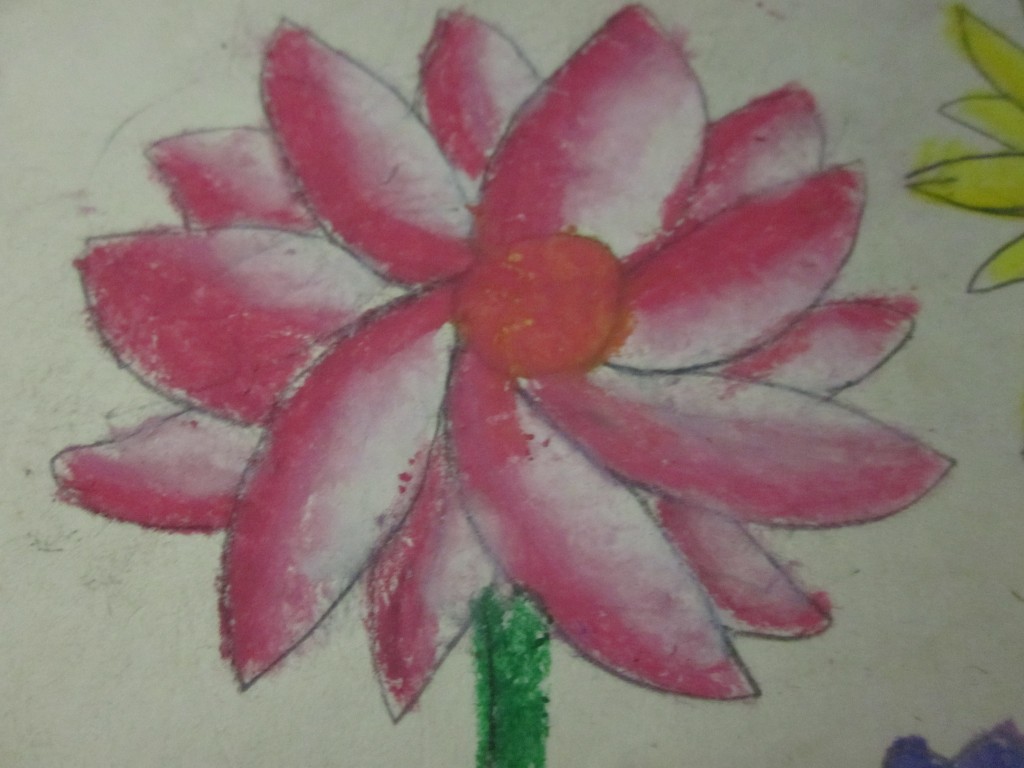The image portrays a meticulously detailed, color drawing of a pink flower on white paper. The outlines of the flower are delicately rendered in either pencil or thin pen, adding a well-defined structure that is subsequently colored in with pastel sticks or potentially watercolor paint. The flower features a round, dark pink center, from which layers of petals emerge. Each petal transitions gracefully from a deep pink at the base, to lighter pink, and finally to white at the tips, creating a soft, blended gradient effect. The flower's bright green stem extends straight downward, providing a vivid contrast to the pink hues. Additionally, the upper right-hand corner of the drawing includes a partial view of another flower—this time with four yellow petals. These slender petals have pointed tips, although the rest of this yellow flower is cropped out of the image.